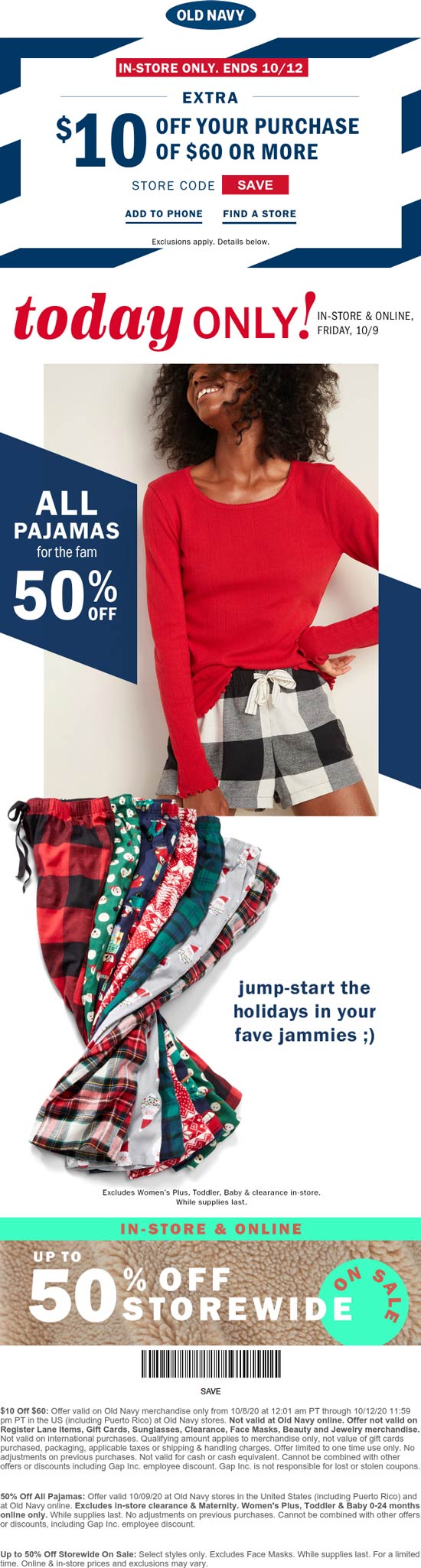This vibrant Old Navy advertisement prominently features the brand name "Old Navy" at the top. Below, a visually striking coupon is highlighted with a blue outlined rectangle that is intermittently broken. The coupon banner at the top is red with white writing that states "In-Store Only, Ends 10-12". Inside the rectangle, a gray line separates the text that reads “Extra $10 off your purchase of $60 or more.” Additional instructions such as "Store Code," "Save," "Add to Phone," and "Find a Store" are visible, along with a note indicating "Exclusions Apply" and "Details Below."

Taking center stage is an announcement for a limited-time offer: "Today Only - In-Store and Online Friday 10/9," with "Today Only" being prominently enlarged and colored in red. Scattered around this announcement are images of various pajama bottoms adorned with festive Christmas motifs. A stylish Black woman with a voluminous afro, modeling black and white plaid shorts paired with a red long-sleeve t-shirt, personifies the offer slogan, "Jumpstart the Holidays in Your Fav Jammies."

Below this visual, another coupon emphasizes an "In-Store and Online" deal offering up to 50% off store-wide with a barcode centered beneath the text that reads "Save". The lower part of the coupon is densely packed with terms and conditions for the $10 off $60 offer. The entire ad is festive and inviting, capturing the holiday spirit and enticing customers with significant savings and limited-time offers.